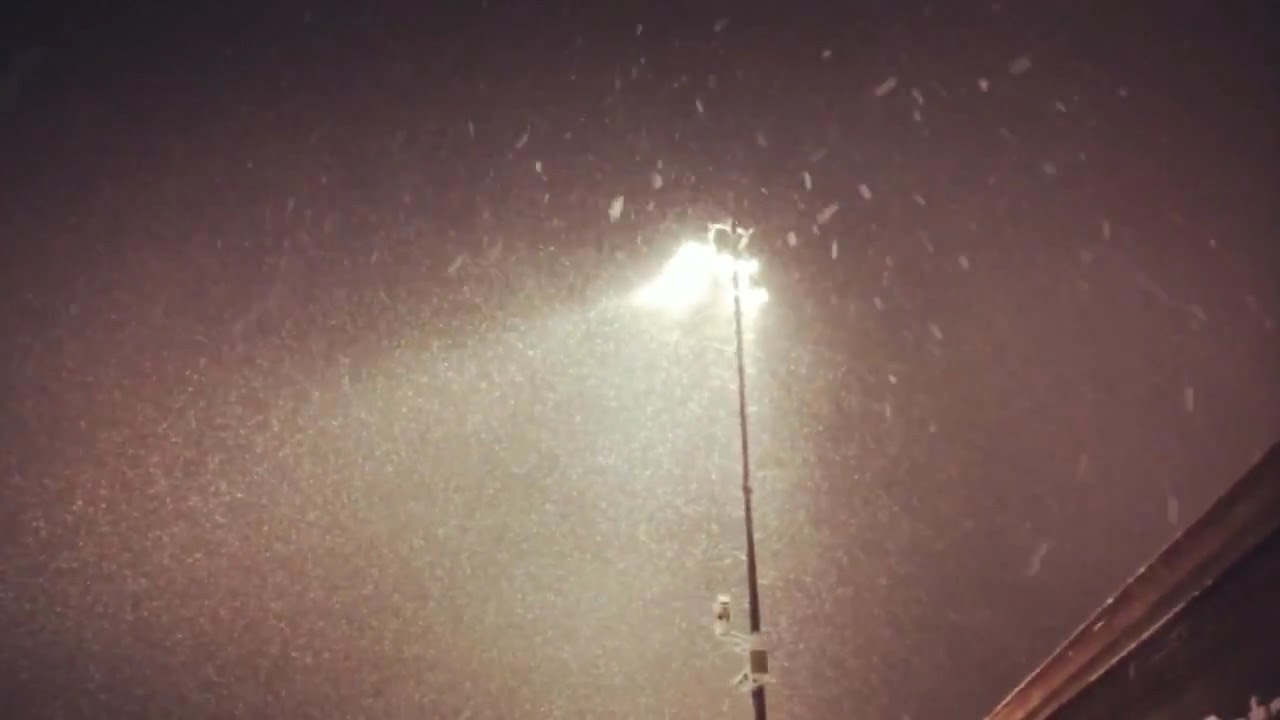The image portrays a dimly lit snowy night, dominated by a black or very dark rock-like object that occupies the center and slightly right portion of the frame. The rock, potentially part of a street light or a stadium light, has an erratic flame at its top, emitting sparks and burning towards the 8 o'clock direction, surrounded by specks of material that reflect the faint light. Snowflakes sprinkle the air, contributing to the scene’s overall diffused lighting and chilly ambiance. A white string-like attachment is noticeable near the bottom of the pole-like structure. To the right, hints of a linear structure, likely the underside of a roof with a distinct brown line, add an architectural element. The dark edges of the image emphasize the nighttime setting, with light from the pole reflecting off nearby snowflakes, creating an ethereal glow amidst the storm.